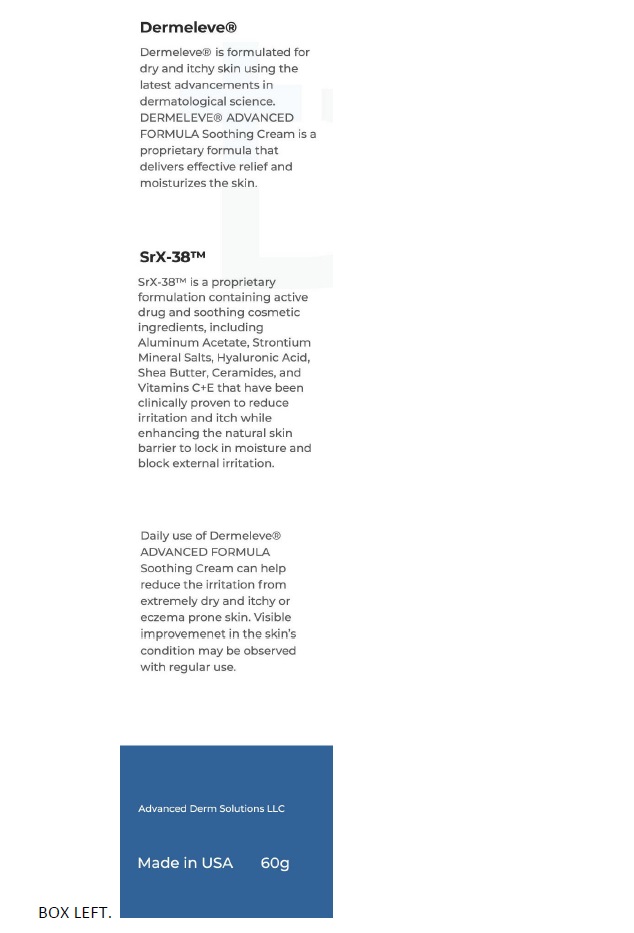A smartphone captures a narrow shot of a product label focusing on Dermaleve® Advanced Formula Soothing Cream, a moisturizing lotion specifically formulated for dry and itchy skin. Utilizing the latest advancements in dermatological science, this cream promises effective relief and enhanced skin hydration. The formula boasts a proprietary blend named SRX-38™, which includes a combination of active drug and soothing cosmetic ingredients such as aluminum acetate, strontium mineral salts, hyaluronic acid, shea butter, ceramides, and vitamins C and E. These components are clinically proven to alleviate irritation and itching while improving the skin's natural barrier to lock in moisture and block external irritants.

Moreover, the label emphasizes that daily use of Dermaleve® Advanced Formula Soothing Cream can significantly reduce skin irritation, especially in individuals with extremely dry, itchy, or eczema-prone skin. Regular application can lead to visible improvements in skin condition.

The bottom of the label features information about the manufacturer, "Advanced Derm Solutions, LLC", highlighting that the product is made in the USA and comes in a 60-gram size. The overall design includes a blue square at the bottom, with text indicating "box left" alongside a dot, suggesting this is a printed template for packaging.